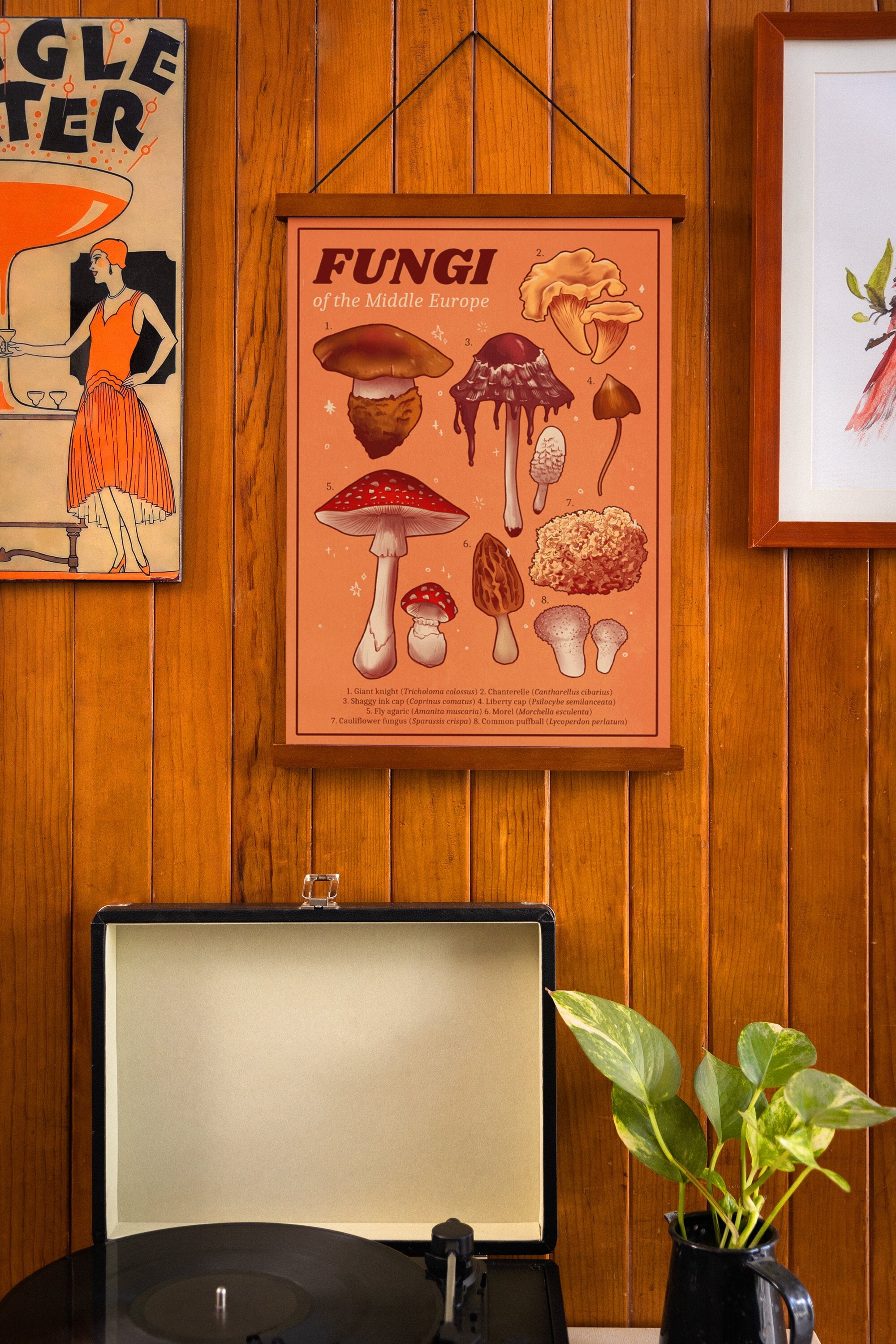The photograph captures a cozy segment of someone's living room adorned with wooden walls of a medium honey color. Central to the image is a framed picture titled "Fungi of Middle Europe," displaying various types of mushrooms on a wooden board. To the left, partially visible, is a vintage-style poster of a 1920s flapper woman in an orange dress, holding a large champagne glass filled with an orange liquid. Another indistinct watercolor painting is slightly visible to the right. Below these pictures sits an open, foldable record player with a record in standby mode. Adjacent to it, a small pitcher, repurposed as a pot, nurtures a green plant with five broad leaves, adding a touch of life to the quaint scene. The combination of these elements on the wooden backdrop offers a warm, nostalgic ambiance.